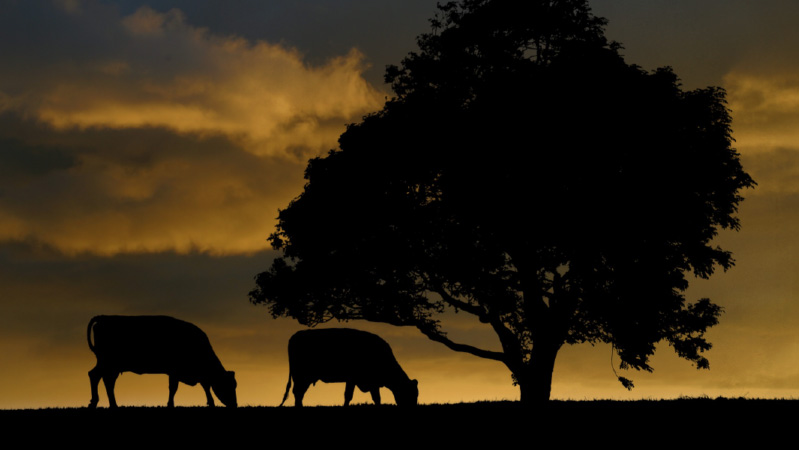This digital photograph captures a serene evening landscape, moments after sunset, with the sun completely below the horizon. The sky is a breathtaking display of different shades of yellow, orange, and red, accentuated by fluffy white clouds scattered primarily on the left side of the image. The setting sun casts the entire foreground into a dark silhouette. Dominating the scene is a large, robust tree with dense foliage, standing almost in the center-right of the image. Close to this tree, there are two silhouettes of cows, positioned one behind the other, oriented so that their hind legs face left and their heads face right. The cows appear to be grazing the grass, which, like the rest of the ground, is rendered in pitch black due to the low light conditions when the photo was taken.